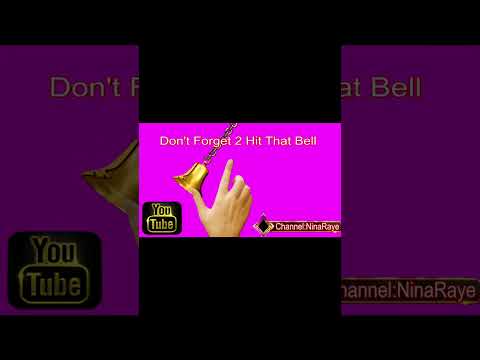The image is a computer-generated representation of an older version of YouTube, set against a black background. The primary focus in the middle features a blown-up, high-contrast webpage showing a YouTube homepage with four rows of six videos each, exhibiting content like CNN Alert and possibly Nina Reyes. Dominating this central section is a large, silver, three-dimensional number 9. Surrounding this are mirrored, darkened images of a YouTube webpage on the left and right sides, faded to the point where they appear almost blacked out. At the bottom of the central image, the YouTube logo is visible, with "tube" in white font inside a red box, though it's distorted and appears mirrored or backwards. Black horizontal bars run across the top and bottom, enhancing the dark, reflective composition of the whole image.